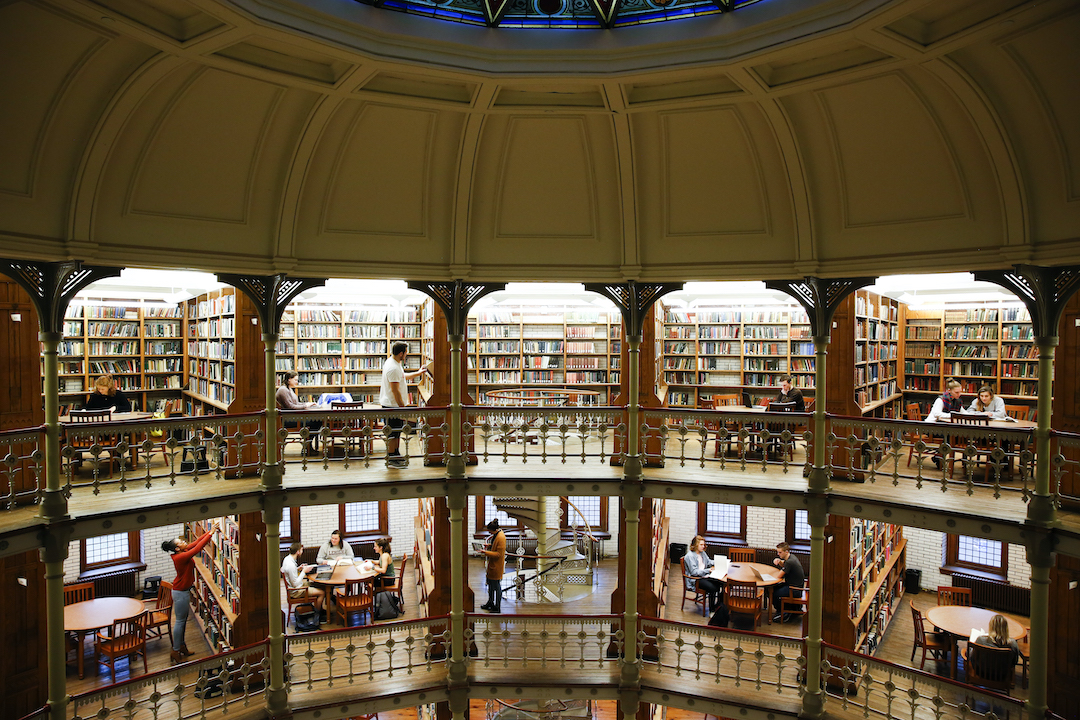This color photograph captures the stunning interior of a rotunda within a library at Lehigh University. The image is taken from the upper floor, looking down into the large, open space. The library features an impressive domed roof with a skylight at the top, allowing natural light to flood the area. The design showcases two visible levels, each arranged around the circular railing of the rotunda and separated by supporting columns. 

The top floor, akin to a balcony, is lined with multiple sections of fully stacked bookshelves and tables positioned for studying. Below, the second floor mirrors this setup, with bookshelves along the walls and designated areas for seating and studying. Several people are seen utilizing the space; a few are seated around tables on the lower level, while one individual is spotted reaching up to a bookshelf. Notably, the second floor also features windows that limit the placement of bookshelves to the sides, offering a picturesque view outside. The architectural elegance is further accentuated by a central spiral staircase, adding to the grandeur of this academic haven. The photograph, with its detailed composition, embodies the essence of photographic representational realism.